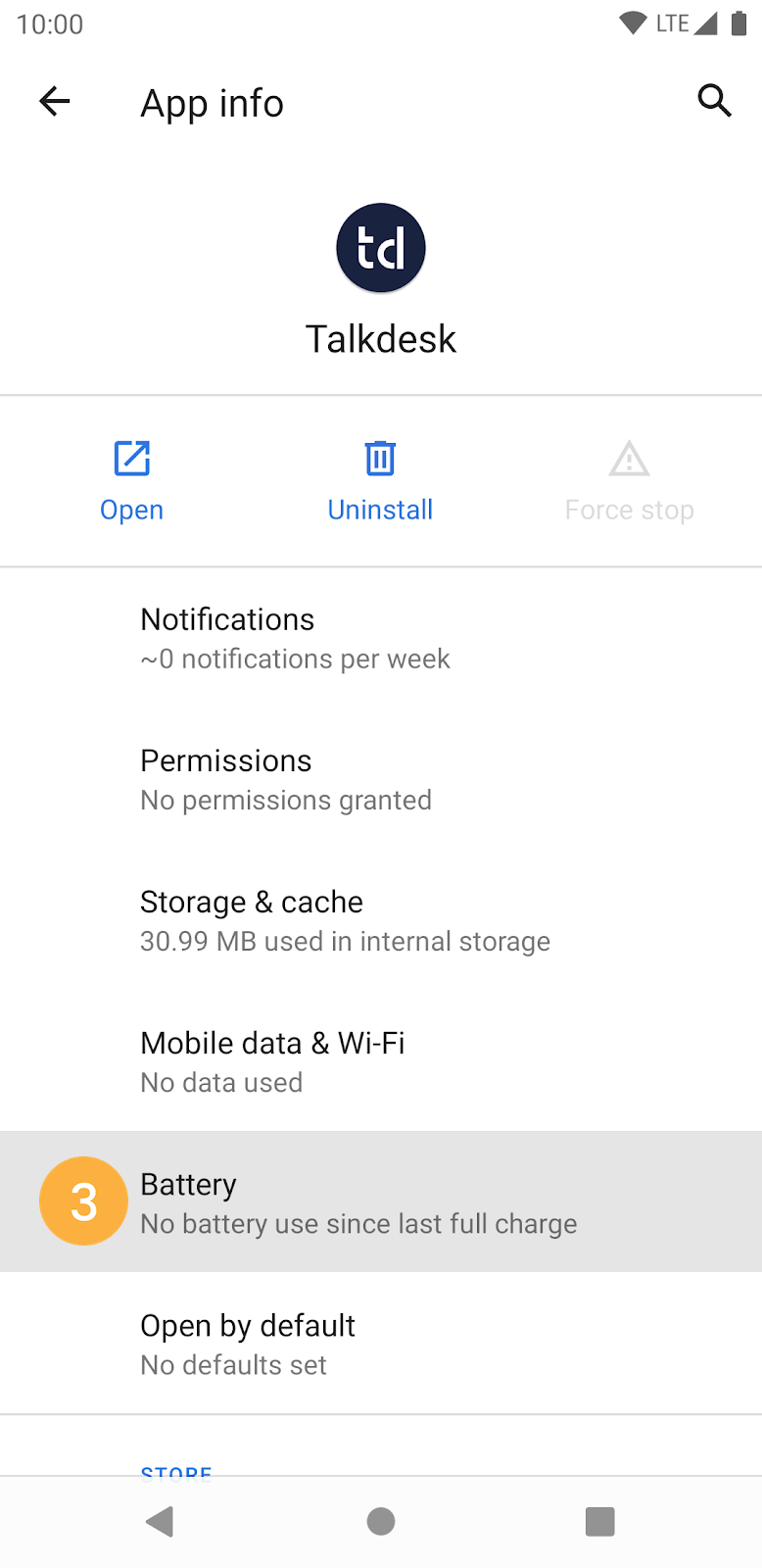Here is a cleaned-up and detailed caption for the given image:

---

**Screenshot of Mobile Device Displaying App Information Page for TalkDesk**

This image is a screenshot taken from a mobile device, likely an Android, displaying the app information page for the TalkDesk application. The device's status bar at the top shows it's 10 o'clock on the left side, and on the right side, icons for Wi-Fi, LTE, mobile data signal strength, and battery status are visible.

At the top of the screen, the header reads "App info" flanked by a left-pointing arrow and a magnifying glass icon. Below this header, there is the TalkDesk logo, which features lowercase letters "t" and "d". Following the logo, three options are presented: "Open", "Uninstall", and "Force Stop", with the "Force Stop" option grayed out, indicating it is not selectable. The "Open" and "Uninstall" options are highlighted in blue.

Further down the page, several expandable sections are listed:

1. **Notifications:** Displays "~0 notifications per week."
2. **Permissions:** Indicates "No permissions granted."
3. **Storage & Cache:** Shows "30.99 MB used in internal storage."
4. **Mobile Data & Wi-Fi:** Indicates "No data used."
5. **Battery:** States "No battery used since last full charge."
6. **Open by Default:** States "No default set."

At the bottom of the screen, there is a blue button labeled "Store." The device's navigation bar at the bottom includes a left-pointing triangle, a circle, and a square on the right, typical of Android devices. Additionally, a small yellow "3" icon is displayed next to the "Battery" heading, potentially denoting notifications or updates related to the battery section.

---